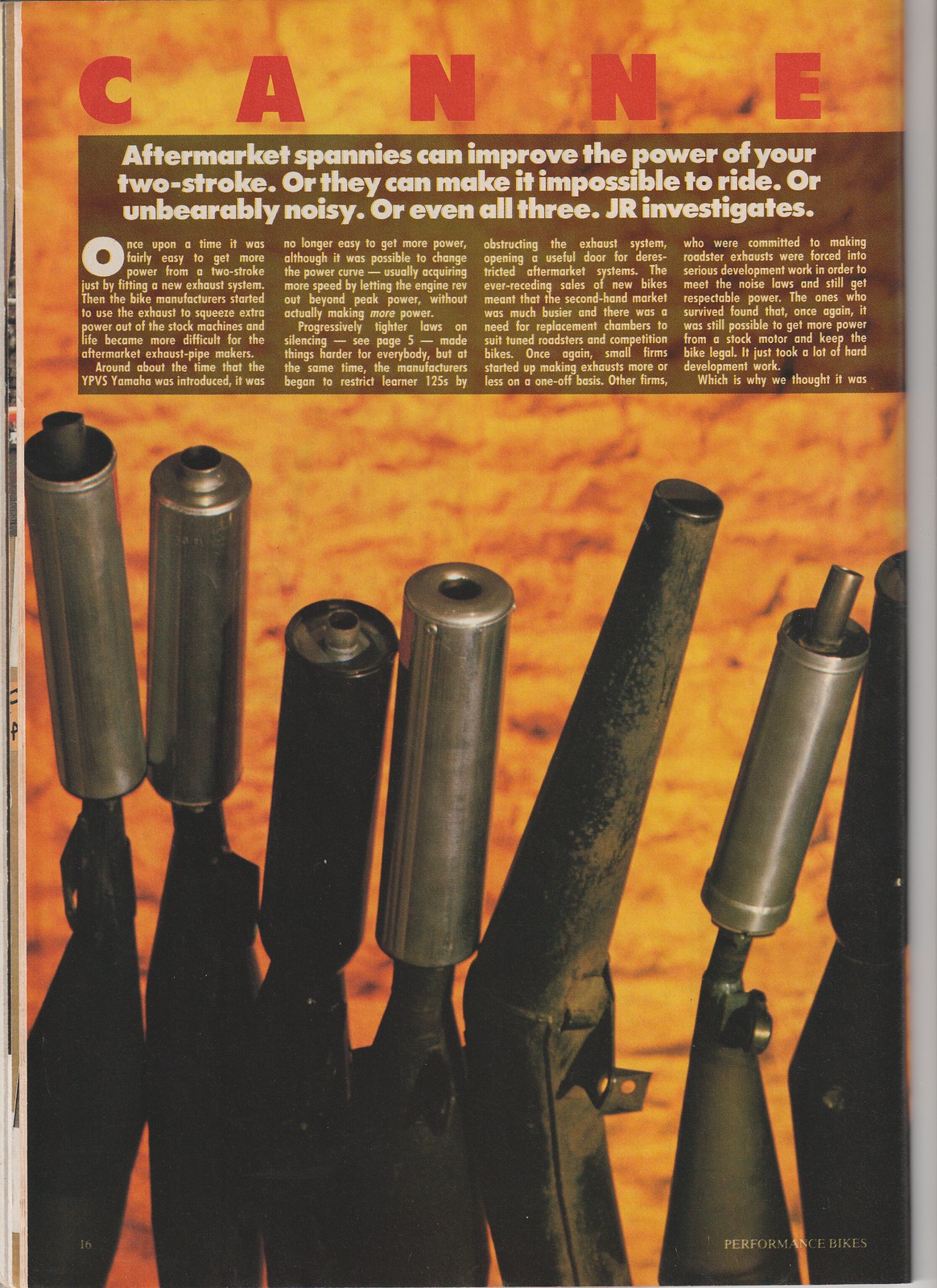The image depicts a magazine page with a bright, textured orange background. At the top of the page, in bold red letters, it reads "CANNE." Below this, in white text, it says, "Aftermarket Spannies Can Improve the Power of Your Two-Stroke, or They Can Make It Impossible to Ride, or Unbearably Noisy, or Even All Three. JR Investigates." The page is filled with an article in four paragraphs discussing this topic. The main visual feature includes several metal devices that resemble tailpipes, primarily cylindrical tubes with one cone-shaped piece. These devices vaguely look like pistols with silencers but are essentially aftermarket parts for two-stroke engines. The detailed page is noted as page 16 of the magazine, labeled "Performance Bikes" at the bottom right corner.